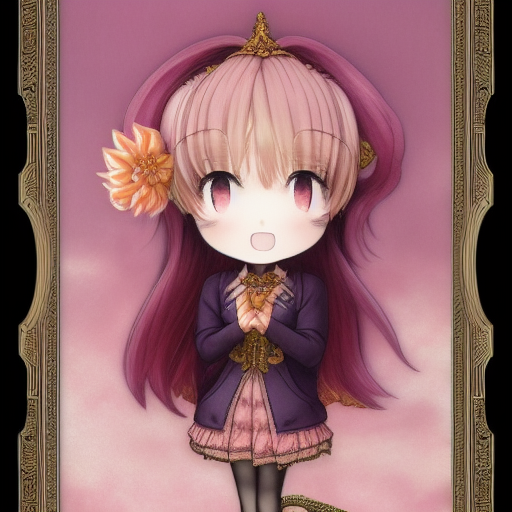This detailed anime art features a central character set against a gradient purple background, transitioning from a darker shade at the top to a lighter hue toward the bottom. The image is encased in a beige frame adorned with intricate line symbol designs. The character, a doll-like anime girl, has long flowing purple hair with white bangs partially covering her wide, oval eyes, which match the darker shade of her hair. Adorned with a gold crown and a peach flower tucked behind her right ear, she exudes a mythical charm. She wears a dark purple jacket fastened at the front with a gold clasp and a gold necklace, over a light purple, nearly pastel-colored dress. Black pantyhose complete her outfit. Her small, pursed lips and open mouth add to her expressive appearance. The very edges of the image feature a black border, enhancing the focus on the vibrant centerpiece.